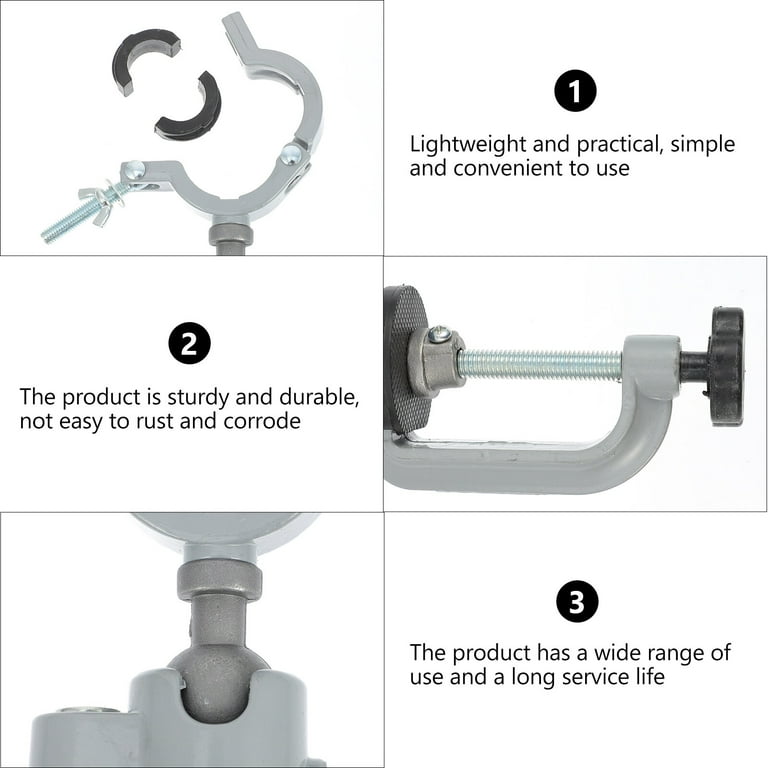The image features three detailed pictures of a specialized mechanical device, most likely a type of clamp designed to securely hold circular or cylindrical objects such as pipes. The device incorporates inserts and a screwing knob mechanism that ensures a firm grip. Accompanied by promotional text, the product is highlighted for its key attributes: 

1. **Lightweight and Practical**: Emphasized for ease of use and portability.
2. **Sturdy and Durable**: Constructed from materials resistant to rust and corrosion, ensuring longevity.
3. **Wide Range of Use and Long Service Life**: Versatile in application, suited for various tasks, and built to last.

The assembly likely includes silver and gray components with black accents, such as the turning handle, which is consistent across all three visual representations. The device features a swivel ball joint on one end, enabling flexible positioning, and is compared to a C-clamp but with specialized inserts that suggest it is designed for particular, not general, applications. Each picture illustrates different stages or parts of the clamp, portraying its robust construction and multifunctional use.